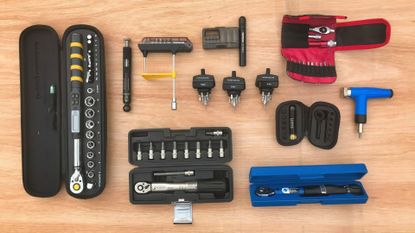This bird's eye view image showcases a meticulously organized assortment of tools laid out on a light wooden table. On the far left, there is a long, thin silver wrench with a black and yellow striped handle housed in an oblong black case. Beside it lies a pencil-like black tool and an oddly shaped black tool. Below these are various drill bit attachments with black holders and silver drill parts. A black case at the bottom contains a silver tool with a black handle, likely accommodating additional drill bits. In the middle, there's a blue case with an unidentified tool and a blue handled tool outside the case. On the top right, a red cloth pouch with black accents holds three small tools, resembling a compact tool kit. Various attachments, possibly for a screwdriver, are lined up across the top right segment of the image. The overall collection is primarily black in color, with notable pops of blue from the cases and the blue handled tool, and red from the cloth pouch with velcro closure.